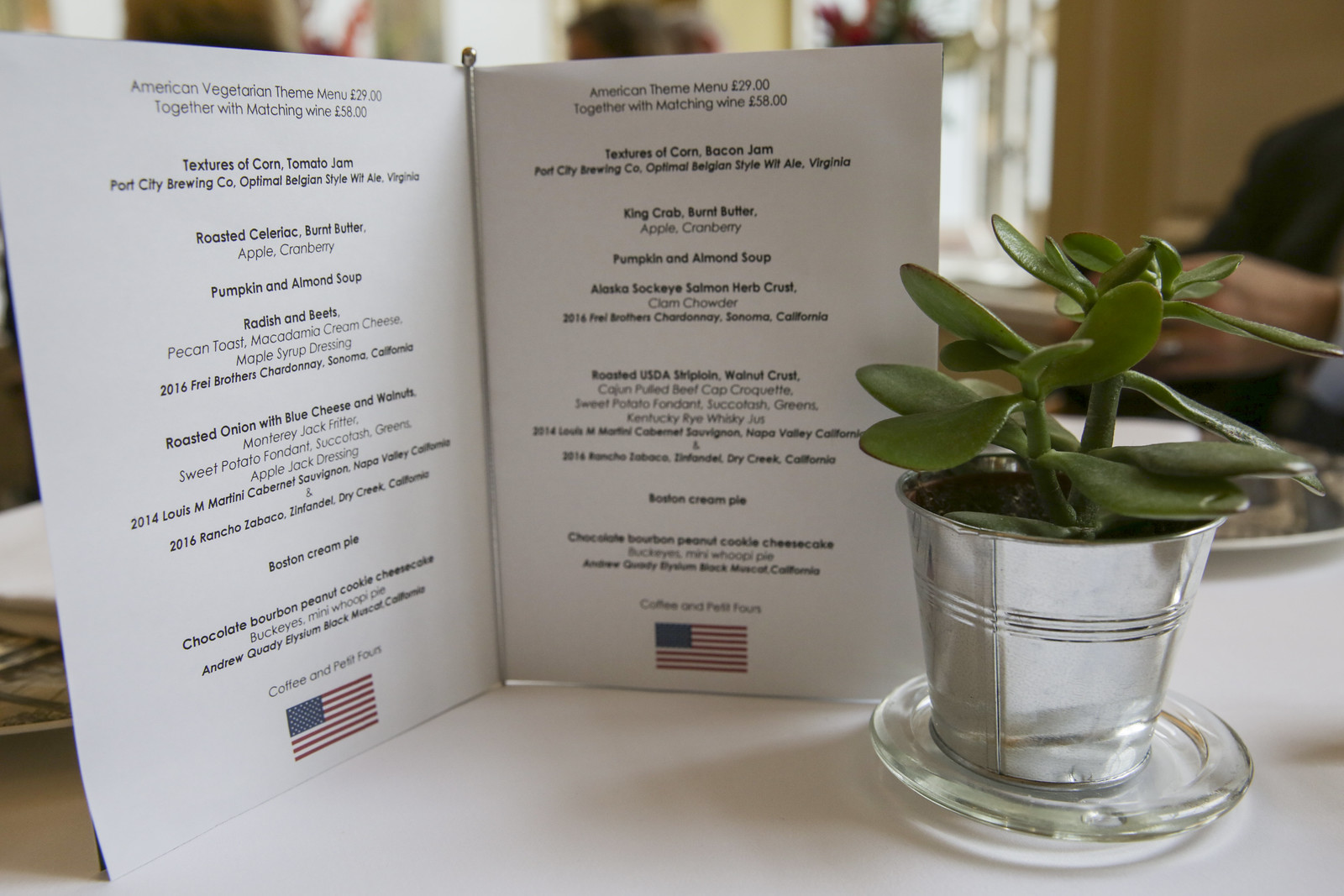In this brightly lit room, sunlight streams through large windows in the background, casting a warm glow over a pristine white table. On the table, an open menu showcases an American vegetarian theme, with dining options priced at 29 pounds and a matched wine selection for 58 pounds. The menu features a variety of dishes including "textures of corn," "tomato jam," "Port City Brewing Company roasted celeriac," "burnt butter pumpkin and almond soup," "radish and beets," "roasted onion," "blue cheese," and "walnuts."

At the bottom of the menu, the American flag is prominently displayed on each side. Beside the menu, a jade plant thrives in a quaint silver pail, sitting atop a round glass coaster designed to catch any excess water. Among the extensive list of menu items are also "textures of corn with bacon and jam," "king crab," "burnt butter," "pumpkin and almond soup," and "Alaska salmon," though some details become unclear as they fade into the page.